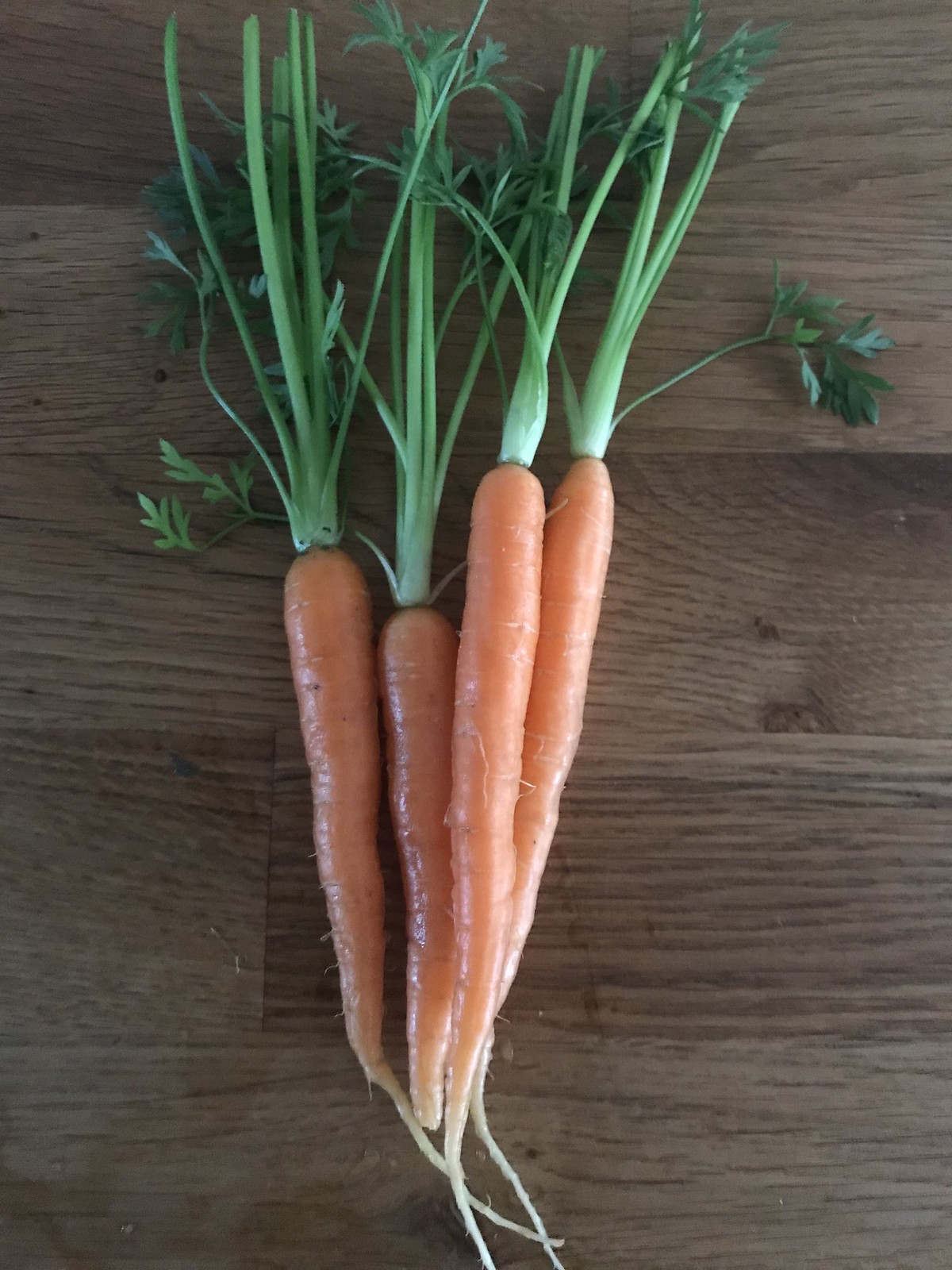This is a softly lit, close-up, vertical photograph of four freshly pulled and washed carrots, laid side by side on a medium brown, wood plank table. The carrots, which are uniform in their vibrant orange color, retain their long, white taproots and have most of their white-to-deep-green stems attached, though many leaves have been removed. Small tendril-like hairs are visible sprouting from their bodies. The soft lighting, indicative of natural light from a nearby window, gently highlights the wooden texture and grains of the table, adding to the rustic charm of the composition.